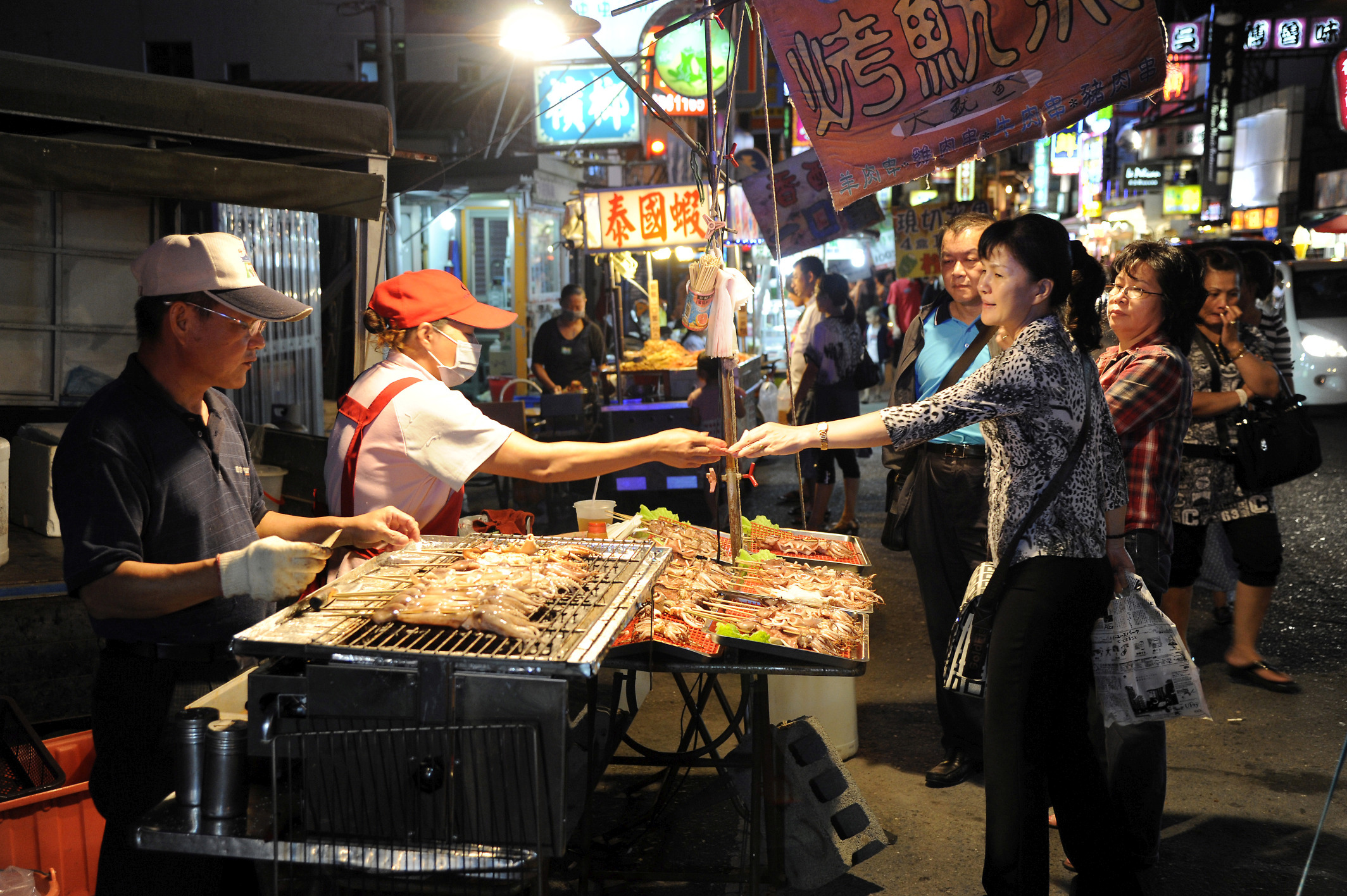In this vibrant photograph set in an Asian locale, likely China, Japan, or Korea, a bustling street vendor scene unfolds against a backdrop of blurred buildings and other vendor carts. At the forefront, a grill laden with skewers of meat takes center stage, releasing aromatic tendrils of smoke into the air. Behind the grill, two individuals work diligently: on the left, a man in a dark polo shirt, glasses, and a baseball cap, dons a white glove on his right hand as he tends to the grill. Beside him, on his left, stands a person in a red baseball cap, white short-sleeved shirt, red apron, and a white face mask, extending their hand over the grill to hand something to a customer—likely completing a transaction. This customer, a woman in a white short-sleeved shirt adorned with black abstract patterns, reaches out with money. She has a black ponytail and short black hair framing her face. Around them, a group of individuals, including a man in a blue shirt and a woman in a plaid shirt, wait in line, presumably deciding on their orders. The scene is vibrant with life as pedestrians mill about and numerous vendor stalls populate the background. Overhead signage with Asian script adds to the authenticity and allure of this busy street market.